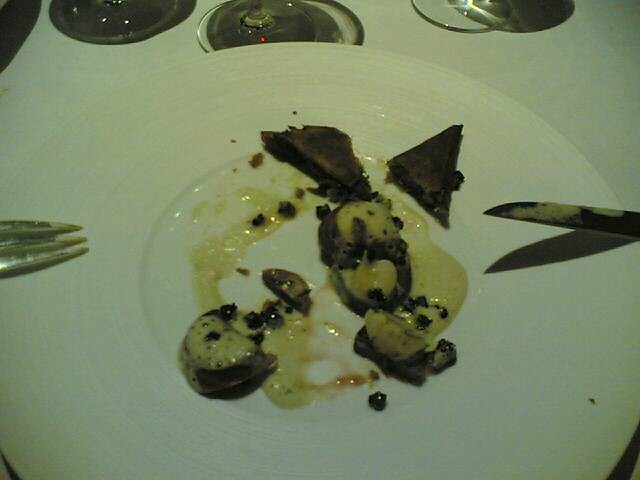In this detailed close-up image, we see a partially eaten appetizer or side dish served on a white porcelain plate, set on a white tablecloth. On the left side of the plate, there's a fork marked with traces of a creamy, yellowish-white sauce, possibly a bechamel. To the right, there are two knives with similar sauce marks. The dish features a small portion of food, indicating it's not a main meal. The central part of the plate holds five morsels: two shaped like triangles and the rest more irregular and chunky. Among these, there are some green vegetables, which could be slices of cucumber, zucchini, or possibly brussels sprouts, and maybe even mushrooms. The precise identity of the dish is unclear, though it might resemble a tandoori-style preparation. At the top of the frame, three wine glasses with thin stems and wide bases are visible, suggesting a fine dining setting.